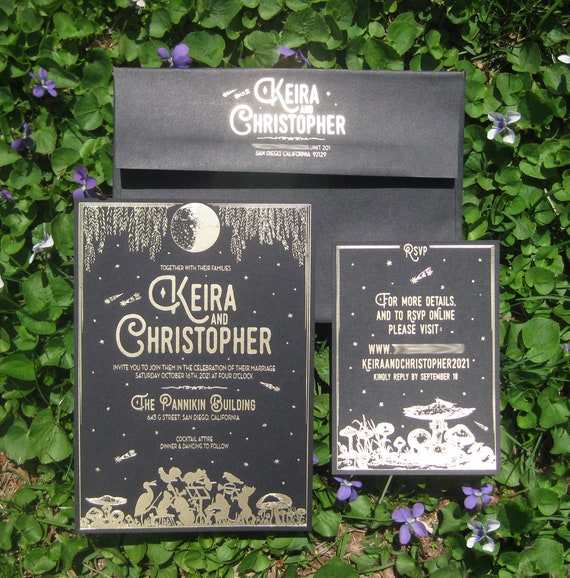This photograph captures an elegant wedding invitation set, thoughtfully arranged outdoors on a lush bed of green ivy adorned with delicate purple flowers. The invitation ensemble comprises three distinct pieces: a larger invitation card, an RSVP card, and a matching envelope, all rendered in sophisticated gray tones with a mix of white and gold lettering.

The backdrop prominently features a dense hedge or a meticulously curated patch of blooming violets, enhancing the natural beauty of the scene. The largest piece, likely the main invitation, occupies the backmost position and features minimalist design elements. Its top edge displays the names "Kiera Christopher" in white, accompanied by smaller, illegible text.

In front of this main card, two smaller gray cards partially overlap it. The left card, showcasing white sprinkles against the gray background, features a central moon image and the names "Kiera and Christopher." It hints at a picturesque setting with silhouetted marine plants or ornamental imagery lining the bottom. Specific venue information, such as the Panikin building, and other minute details affirm the invitation nature while small text remains too fine to discern.

The right card, outlined in white, prominently bears the word "RSVP" and invites guests to get more details and RSVP online, directing them to a mildly blurred URL. This card repeats the names "Kiera and Christopher," framing further instructions for the invitees.

Overall, the composition exudes a meticulous and artistic invitation layout set against a vibrant and natural floral backdrop, signifying the joyous occasion of Kiera and Christopher’s wedding.